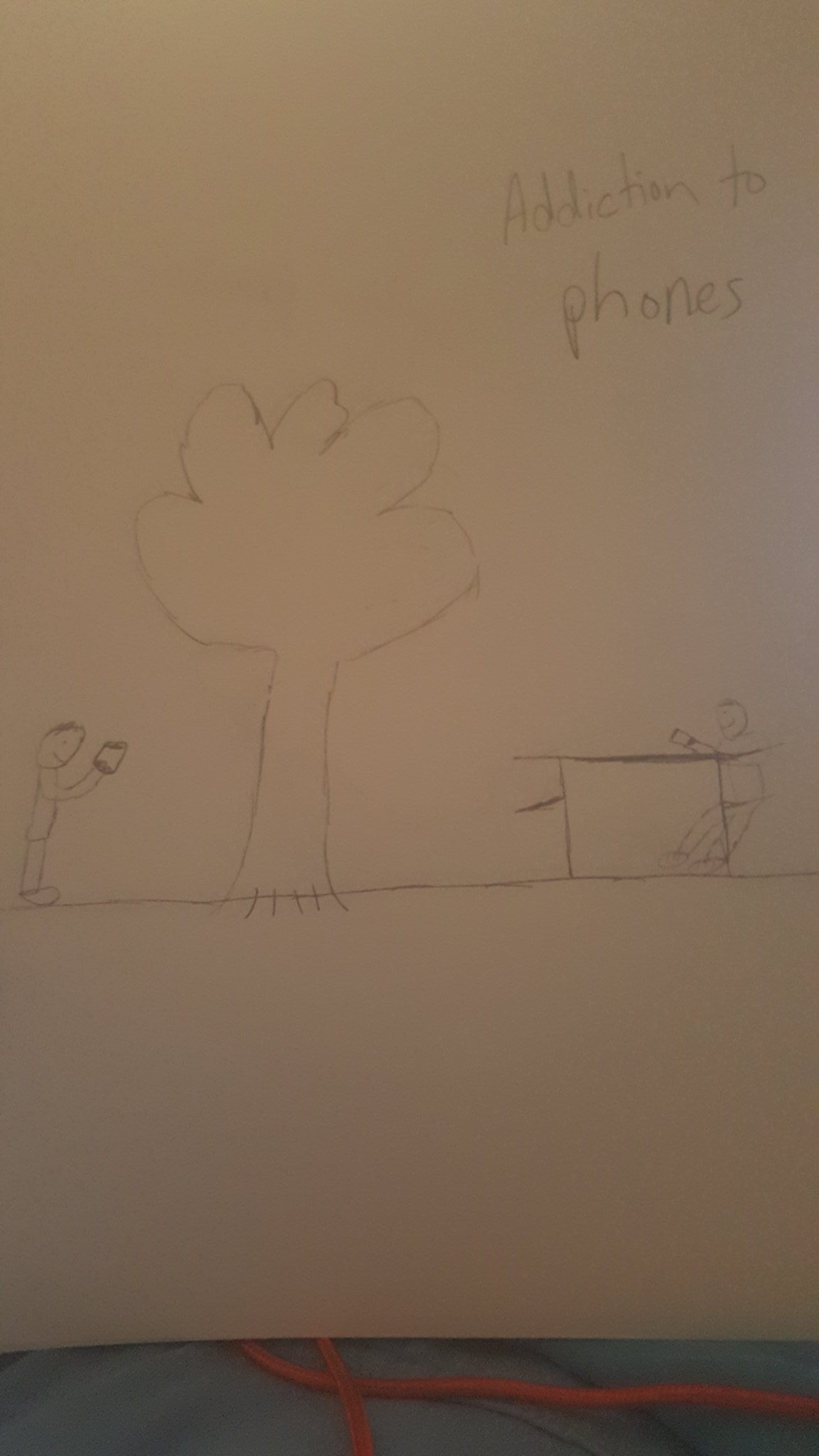This image, though of low quality, appears to be a photograph of a hand-drawn sketch on plain white paper. The sketch, likely done by a child using pencil, depicts a simple yet expressive scene. At the center is a tree with a sturdy trunk and an exaggeratedly fluffy canopy. To the left of the tree stands a figure, presumably male, characterized by a round head and a stick-like body. On the right side of the tree is a table, at which another person is seated. Notably, both figures are holding what appear to be smartphones in their hands. Above the drawing, the artist has scribbled the phrase "Addiction to phones," emphasizing the theme of the illustration. The raw and unrefined style of the elements and the handwritten note suggest a youthful perspective on the subject matter.